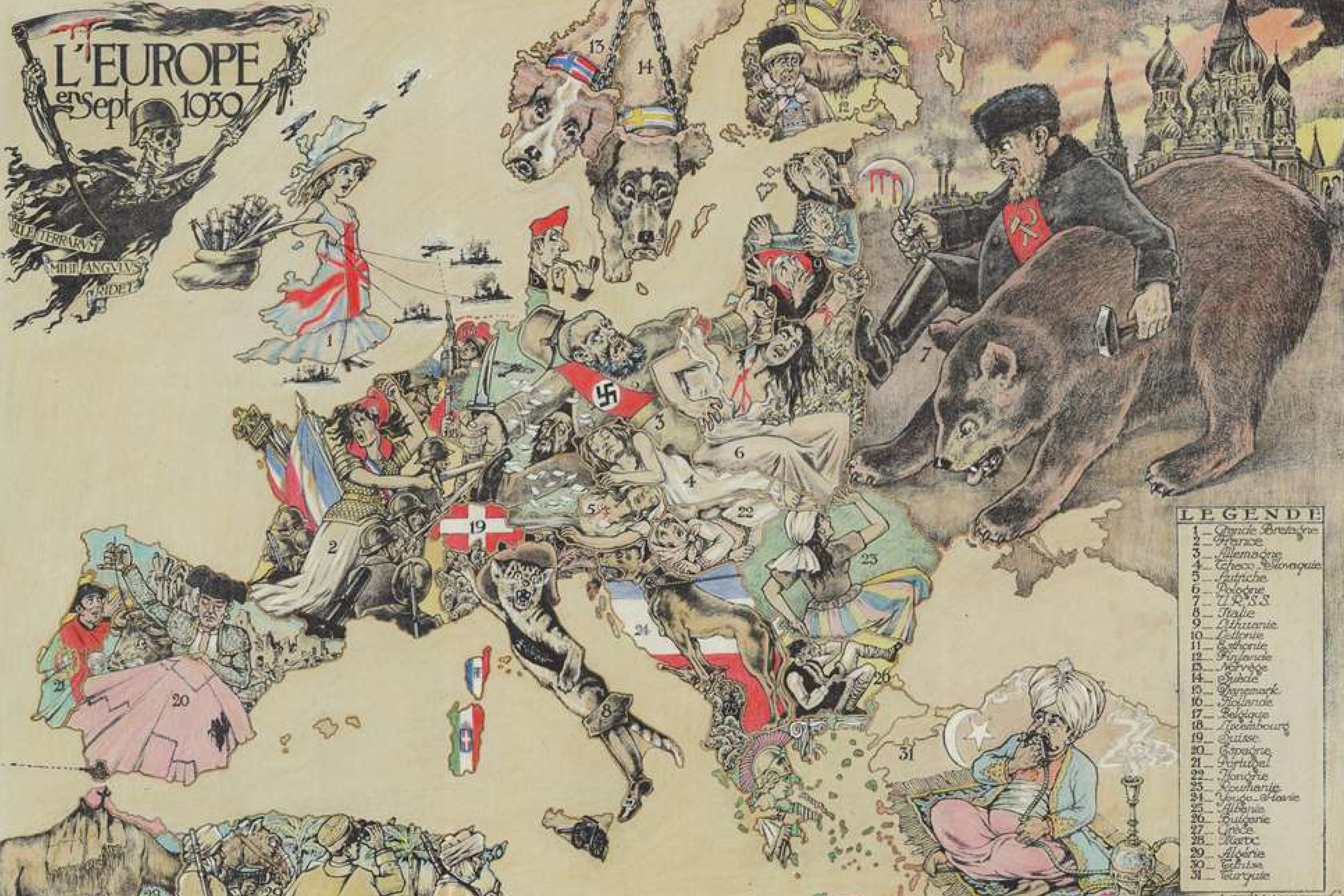This image is an artist's caricature of Europe in September 1939, detailing various country leaders and their actions during the onset of World War II. In the top left corner, a menacing skeleton brandishes a scythe and torch over the continent, with the title "L. Europe" signifying the period. Below this ominous figure, small, unreadable text hints at further context. The map itself is decorated with symbolic characters representing each country: Nazi Germany is depicted committing atrocities under the swastika banner; France, symbolized by a king trying to mend torn fabric, displays its struggle to resist Germany; Britain appears as a woman in a dress resembling the British flag; and Italy, whimsically illustrated as a boot with a jaguar, reflects its unique shape and wartime posture. Russia is shown grappling with a bear, an icon of its power and ongoing battles, and features the Kremlin in the background. To the south, Egypt is illustrated with camels and onlookers amidst the chaos. In the bottom right, a legend numbered 1 to 31 likely corresponds to each nation’s caricature, but the text is too small to discern. Turkey is depicted as a man on a carpet with a turban, gently smoking from a pipe and observing the unfolding events. This richly detailed portrayal captures the tension and turmoil of Europe at the brink of war.